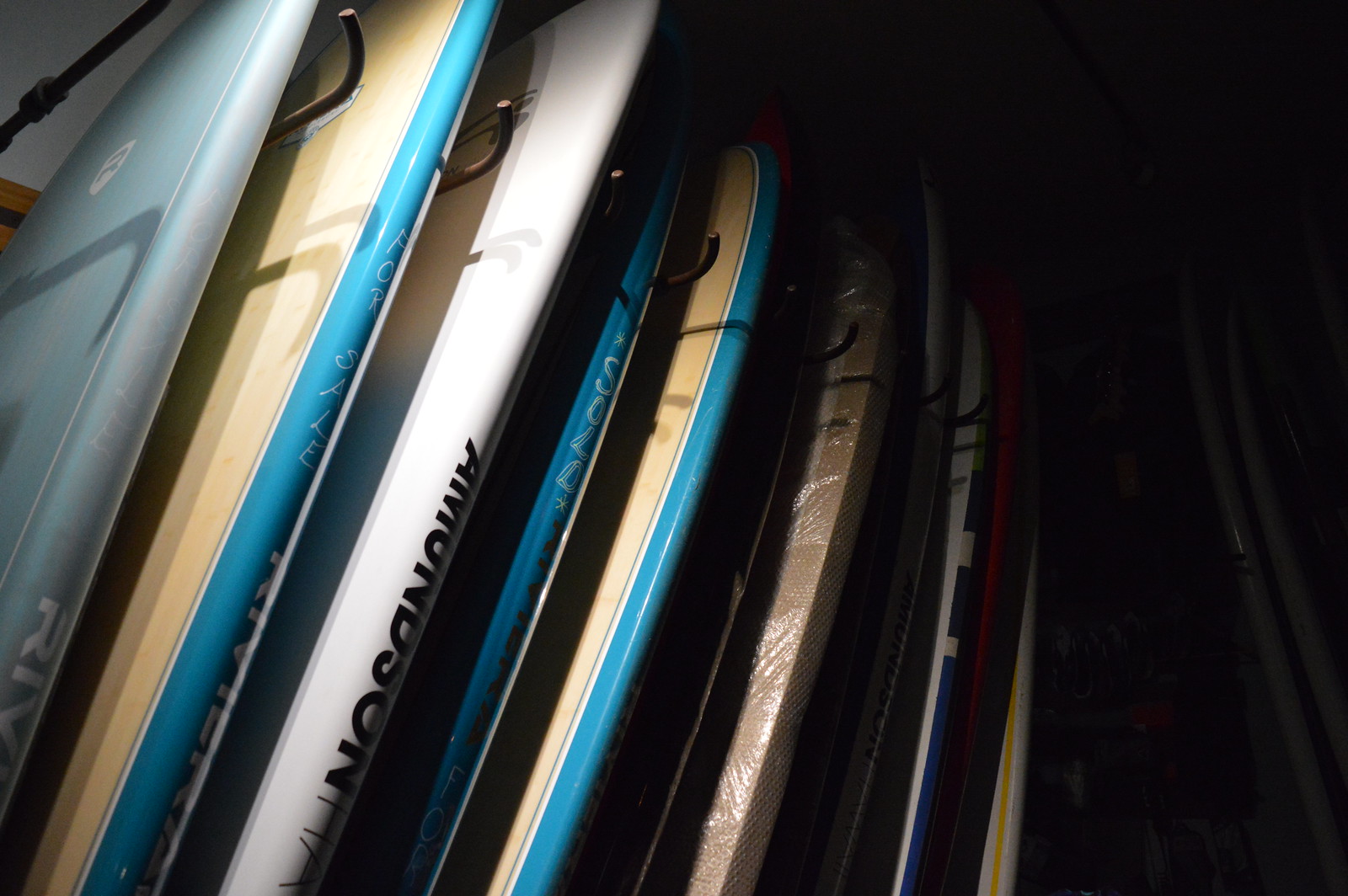This image features a tightly stacked row of approximately ten surfboards leaning against a wall. The photo is a very close-up shot, which makes it challenging to discern the full context, but the distinct shapes at the top confirm they are surfboards. The left side of the image is slightly better illuminated, likely by natural sunlight, revealing some details and colors. The surfboards on the left include a light gray one, a striking teal blue and wood one, another white surfboard, alongside another blue and wood surfboard. Additionally, a pink surfboard is also visible among this group. As the view progresses to the right, the image becomes significantly darker, reducing visibility and merging the surfboards into shadowy outlines without distinct colors. A few hooks and plaque bars can be seen holding the boards in place, but no notable background details are visible. Some surfboards have illegible writing, except a white one that faintly displays “For Sale,” and another with partial black text, “I am on the sun.” Overall, the clustering and dim-lit setup emphasize the spines and edges of these surfboards, giving the impression of a dense, somewhat enigmatic scene.